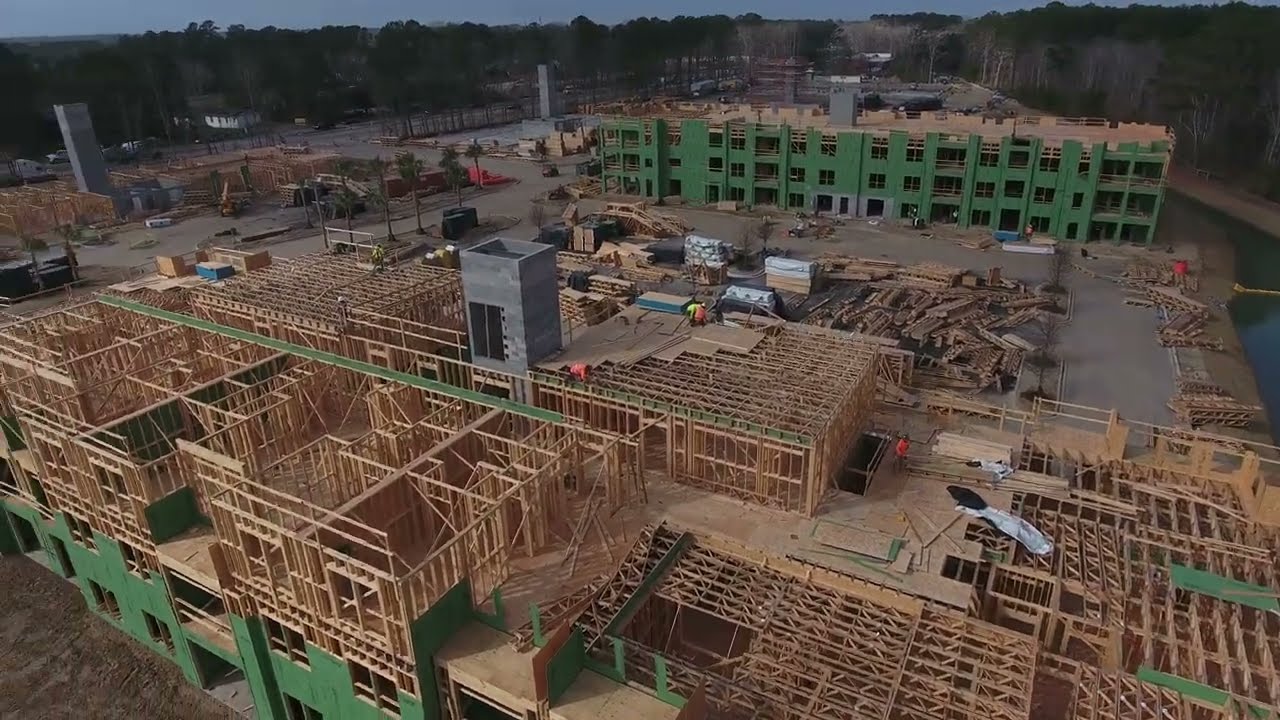The image presents a detailed aerial view of an active construction site for a complex of multi-storied buildings, elevated roughly 50 feet above ground level. The site consists of a set of two rectangular buildings in close proximity, one near the camera and the other further away. Both buildings share a similar design with exposed wooden frames, distinct window openings, and a noticeable green cladding or wrap on some finished sections while others remain framework. The courtyard area between the buildings is filled with construction materials and tools, particularly piled at the center, and bordered by a driveway for easy access. Adjacent to this, another driveway on the left is lined with additional construction equipment. A recurring feature in the image is several stone-like towers or shafts, potentially serving as chimneys or elevator shafts, distributed across the site. The dirt expanse of the construction area is surrounded by trees, adding a touch of nature to the otherwise brownish-toned, debris-laden scene. Amidst the construction chaos, workers can be observed carrying out their tasks.